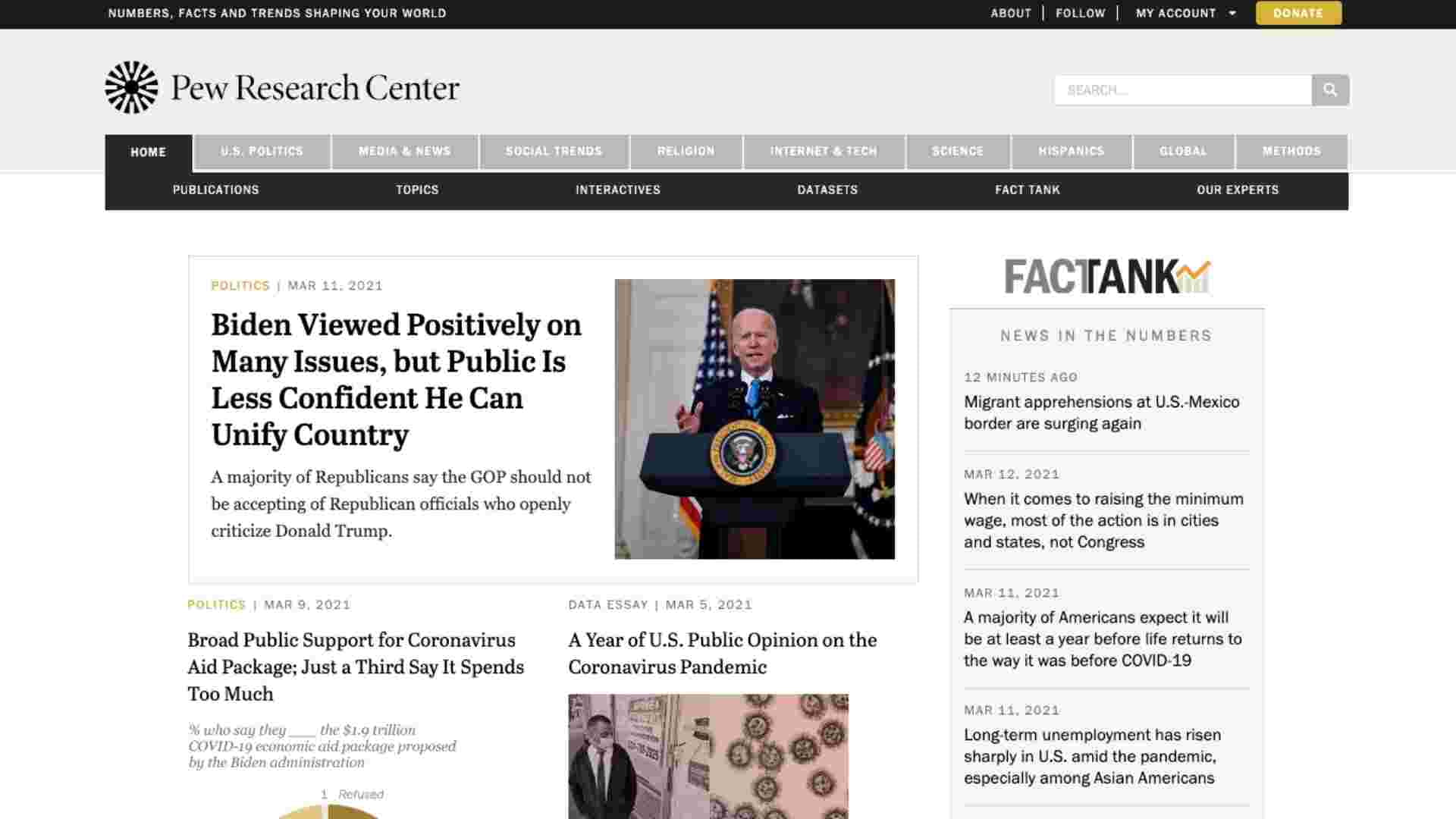Image Caption:   
A collage displaying various recent findings from the Pew Research Center, touching upon the pandemic's impact on political, social, and economic aspects of American life. At the center of the image, a headline notes that President Biden is viewed positively on many issues, although public confidence in national unity remains low. A prominent section to the bottom left highlights broad public support for coronavirus aid packages, particularly in the context of a newly switched state. To the right, data emphasize the differing impacts of the pandemic across Mexican, American, Puerto Rican, and San Diegan populations. Key dates are highlighted: on March 12, 2021, the focus is on raising the minimum wage primarily through local and state actions; on March 11, 2021, Americans express the belief that it will take more than a year for life to return to pre-COVID normalcy, and address the sharp increase in long-term unemployment, especially among Asian Americans. The right side of the fact tank comprises numerical data, visually supported by various branches representing collaborative efforts across the Americas.